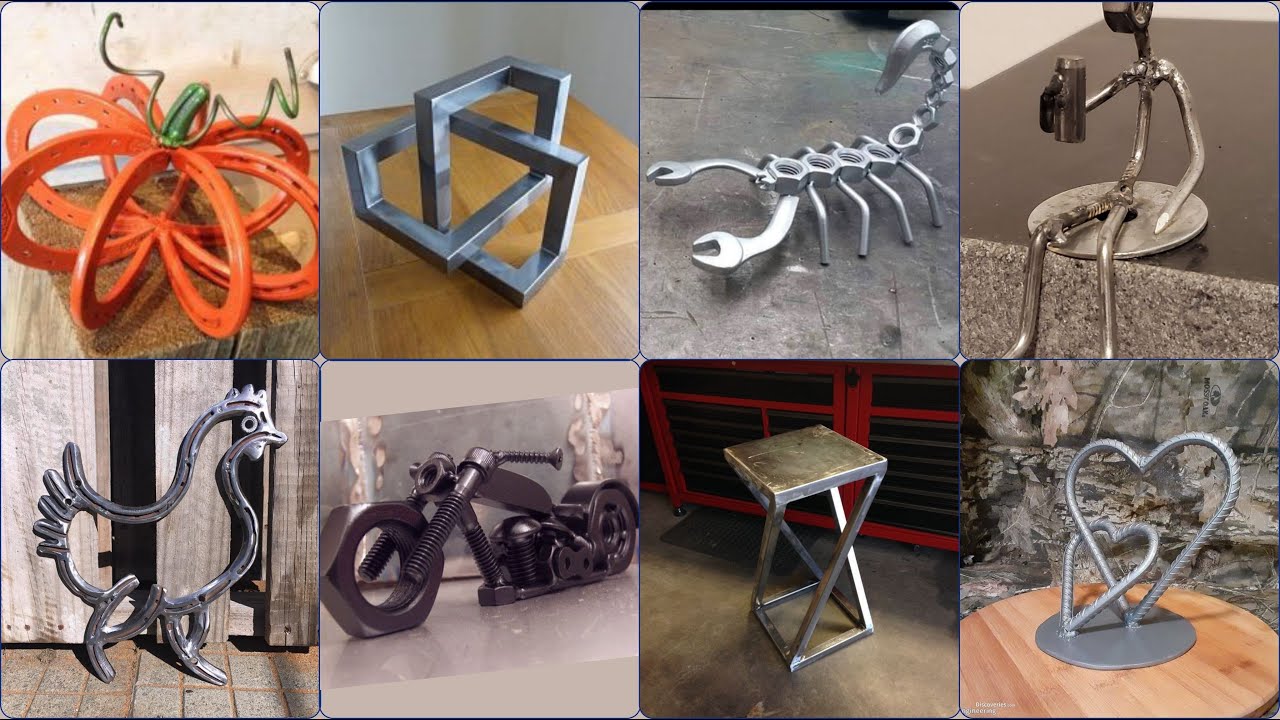This image is a collage of eight distinct metal sculptures, showcasing a diverse range of artistic styles and craftsmanship. Starting from the upper left, we see an orange, wire-frame pumpkin with a green curly stem, potentially crafted from horseshoes and suitable as a lighting fixture. Adjacent to it is a complex silver cube, resembling an intertwined square puzzle. The next photo features an intricate scorpion sculpture created from wrenches, nuts, and bolts. Following this is a wire-frame stick figure sitting on a round base, holding what appears to be a cup of coffee or a travel mug.

Directly beneath the pumpkin, there's a rooster or chicken made from metal, possibly horseshoes, adding a rustic charm. To its right, a detailed motorcycle sculpture is constructed from an assortment of nuts, screws, and bolts. Next is a sleek, silver end table, suggesting a functional art piece. Finally, the last image captures two interlocking hearts made from screws, emphasizing the theme of connection and unity in their metallic form. Each sculpture in this collage beautifully exemplifies the creativity and skill involved in transforming everyday metal objects into unique works of art.